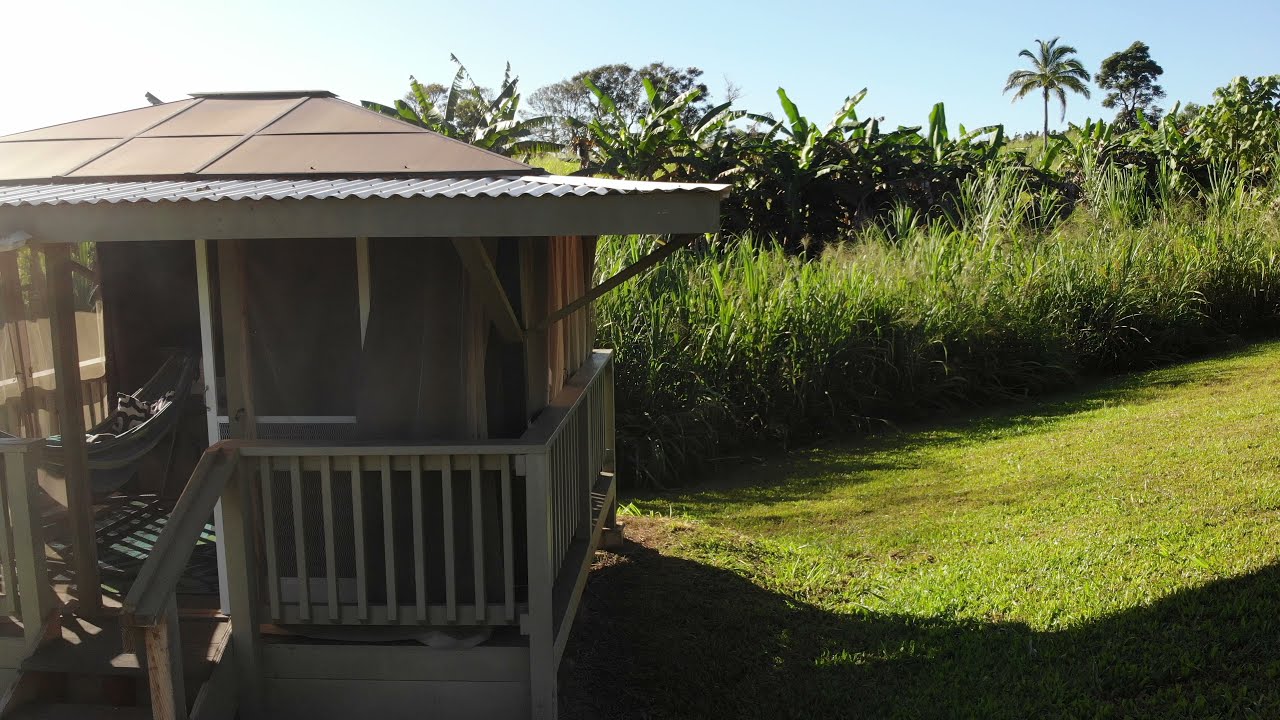The photograph captures a vibrant tropical landscape featuring a small, elevated hut on the left side. The hut, possibly a single-room residence or beach porch, is built on low stilts with a peaked red-tiled roof bordered by an aluminum gutter. The structure is accessed via a wooden staircase with a vertical railing leading to a screened porch. The porch seems to have mesh or curtains for privacy and houses a hammock inside. Surrounding the hut is a lush green grassy hill extending to the right, with sunlight casting a long shadow of the hut onto the lawn. Beyond the grassy area is a dense row of sunlit tropical shrubs, followed by a horizon of tall palm trees and large-leafed trees. The clear, blue sky overhead indicates the photo was taken during a bright sunny day.